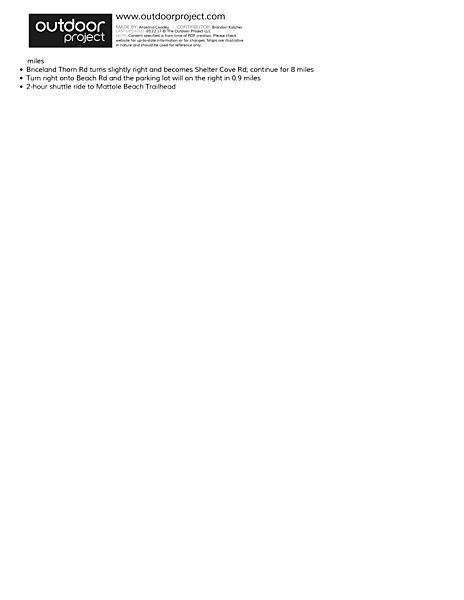The image displays a small segment of a website. In the top left corner, there is a black rectangle with the words "Outdoor Project" written in white. To the right of this, the website address "www.outdoorproject.com" is visible. Below these elements, there is an area containing very small gray and black text, which is mostly illegible even upon zooming in. Additionally, there are three small black text notes arranged vertically. The entirety of the image is set against a white background, giving it a clean and minimalistic appearance.